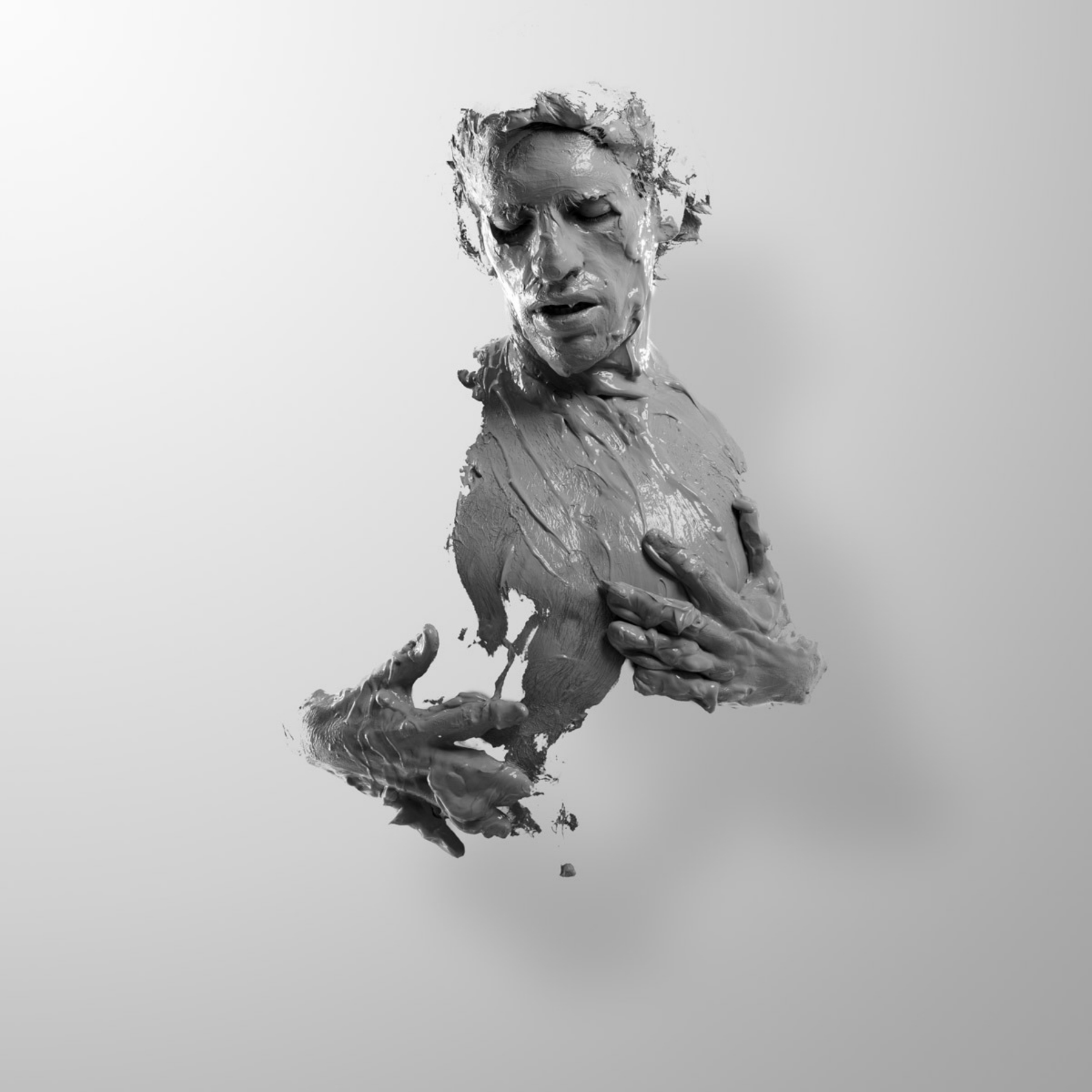The image depicts a surreal, abstract sculpture that combines elements of a human figure with a muddy, clay-like texture. The central focus is a partially visible human figure with a face, chest, and hands seemingly melting and dripping with thick, gray clay. The sculpture appears to be floating against a monochromatic background of grayish-white, creating a stark contrast and emphasizing the emptiness around it. The illusion of parts of the body being tangible is further enhanced by a faint drop shadow, suggesting an advanced technique, possibly involving green screen technology, to isolate and enhance the gray, clay-covered areas. The overall composition is highly detailed yet distinctly abstract, evoking thoughts of muddy volcanic eruptions like those seen in Yellowstone, making it reminiscent of an AI-generated art piece.